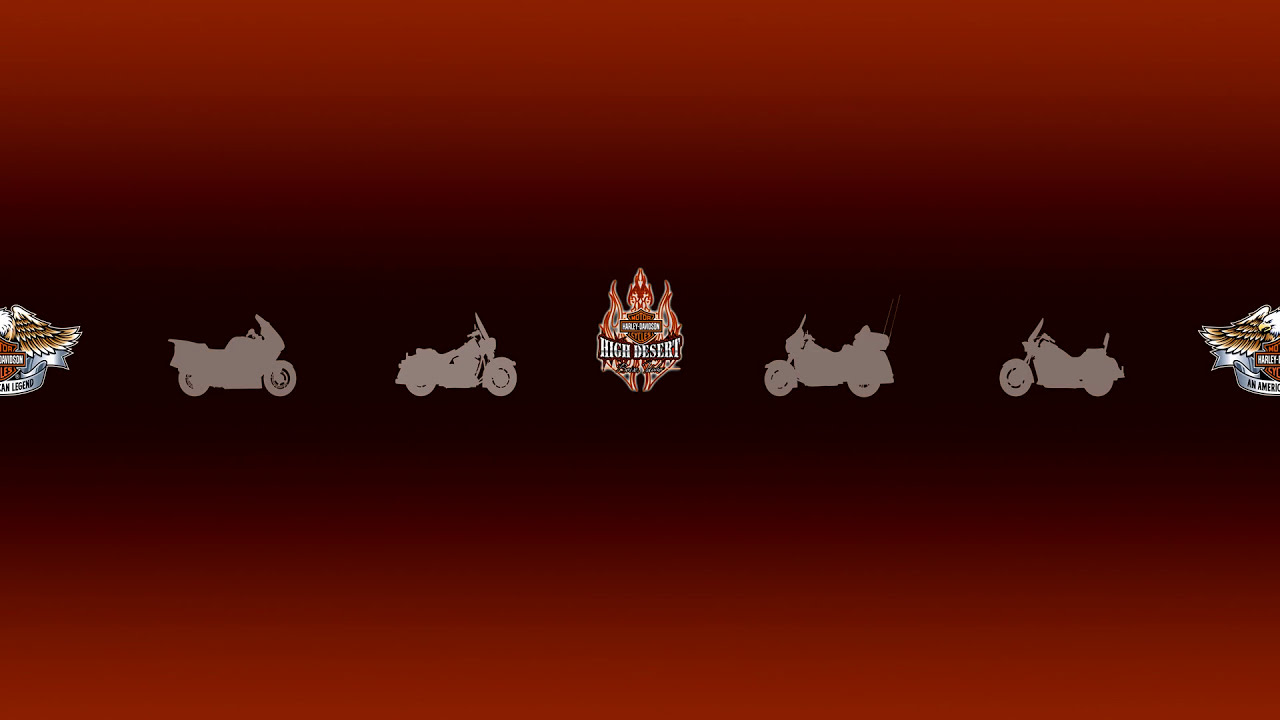This is a detailed and descriptive caption combining the consistent details from the different voices:

This advertisement is a red, horizontal rectangular poster promoting Harley-Davidson motorcycles. The background transitions from a bright red at the top and bottom to black in the center, creating a gradient effect. Across the center of the poster, there are horizontally positioned silhouettes of four different types of motorcycles, all shaded in gray without any additional coloring. On either side of the motorcycles, the Harley-Davidson logo is faintly visible, featuring eagle wings spread out. In the center of the advertisement, there is a distinct logo for 'High Desert,' depicting a figure resembling a Buddha with raised arms, surrounded by a design of flames in yellowish-red hues. The words 'High Desert' are in white with a black border, adding contrast and prominence to the central emblem.